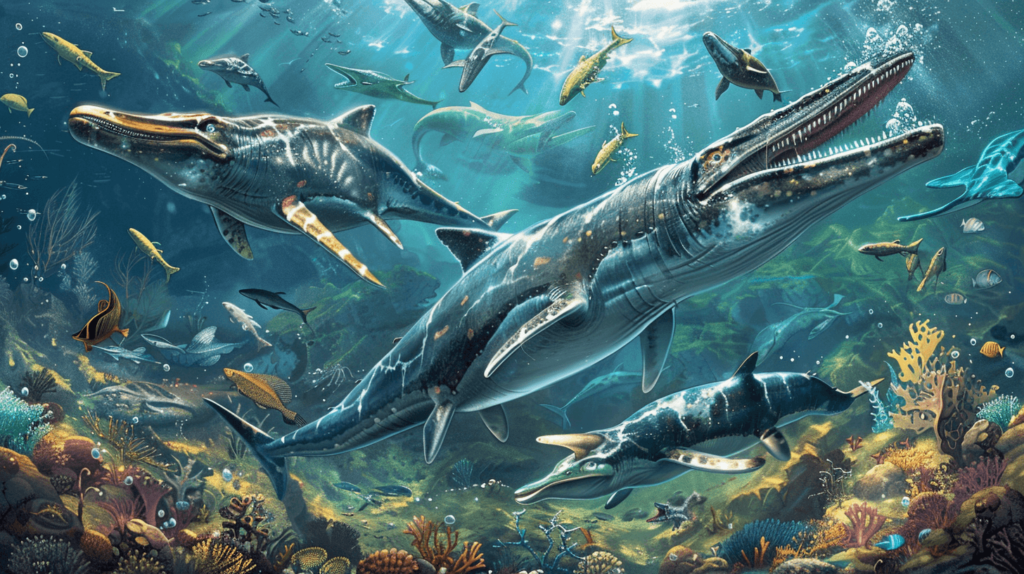This horizontally aligned rectangular artwork is a vibrant and imaginative underwater scene. The perspective is from the ocean floor, looking up towards the surface, where rays of sunlight pierce through greenish-gray water, creating an ethereal backdrop. In the top middle of the image, the sunlight adds a striking effect that resembles feathery clouds. Dominating the center of the image is a large, shark-like creature with an open, pointed mouth filled with small, sharp teeth arranged in a long row. Its narrow tail and prominent dorsal fin enhance its menacing appearance. Surrounding this central figure are various other marine creatures, all uniquely designed in a way that suggests they are more artistic renditions than real-life fish. Some of these additional creatures are smaller sharks, while others are fish of diverse and imaginative shapes and sizes. At the very bottom, the ocean floor is adorned with pretty plants, mostly in brown with some green, and scattered coral, adding to the rich, detailed composition of the scene. The teeming marine life and the surreal quality of the creatures amplify the painting’s artistic allure, making it a visually captivating print.